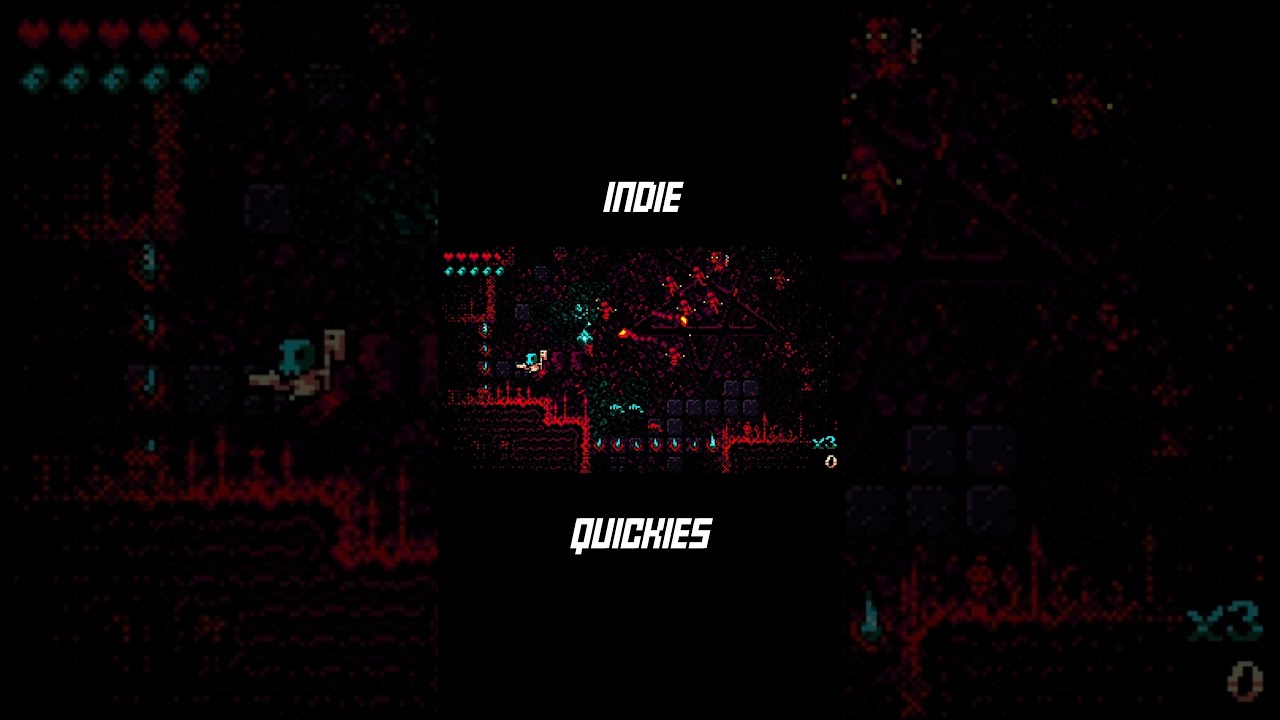In this highly pixelated and dark video game screenshot, the central focus is a small but vivid gameplay image surrounded by a background formed by an enlarged and faded version of the same scene. This creates a distinctive border with prominent black bands at the top and bottom featuring the text "Indie" in white at the top and "Quickies" at the bottom. The gameplay itself shows a tiny, detailed figure with a blue skull-like head and white shirt, wielding a cream-colored ax or gun, navigating a red and black underground environment. This character is pursued by red, skeleton-like enemies shooting fireballs, all while traversing a terrain marked by red outlines, stone tiles, and scattered flames. To the left, a zoomed-in view highlights the blue-headed character, while the right side shows an up-close view of the red enemies. The dimly lit border helps alleviate the dark theme while adding a layer of depth and detail to the scene, and in the bottom right corner, the text "X3" and "0" are visible, possibly indicating a score or remaining lives.